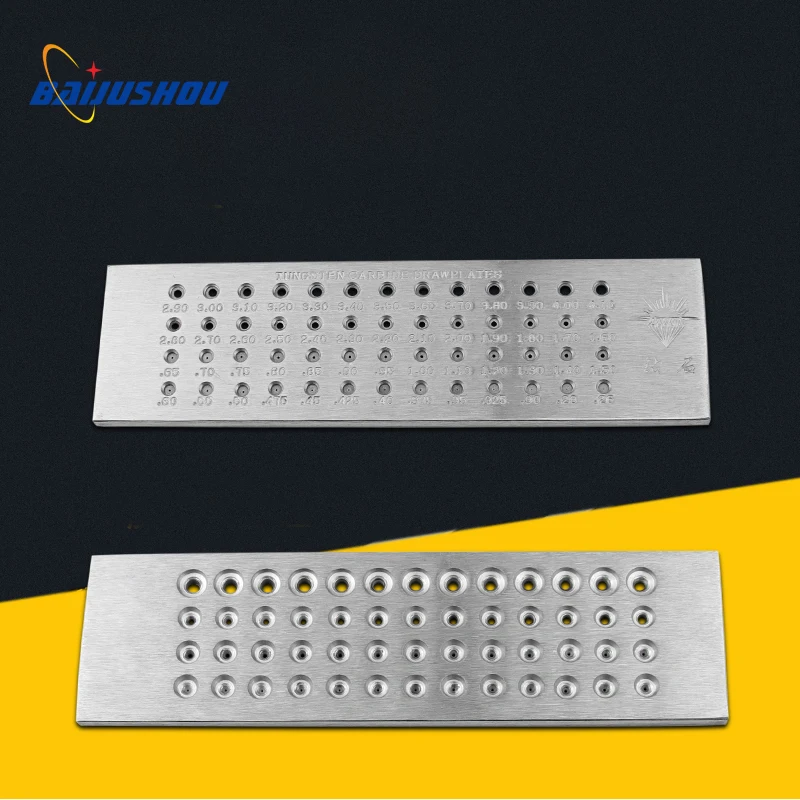The image depicts two metal plates, presumably showing the front and back of a single rectangular draw plate made of tungsten carbide. These plates have a brushed metal appearance and are punctuated with a total of 48 circular holes arranged in a grid of 12 rows with 4 holes each. The holes vary in diameter, starting larger and progressively getting smaller, each clearly marked with corresponding numbers. The largest visible diameter is 9.0, and while some numbers aren't legible, others include 2.90, 3.00, 3.10, and so forth. At the top of the plate, the words "tungsten carbide draw plates" are engraved, and the product branding, "Baiju Show," is showcased in a blue font encircled by a gold halo, positioned on a black and yellow background with a red star detail.